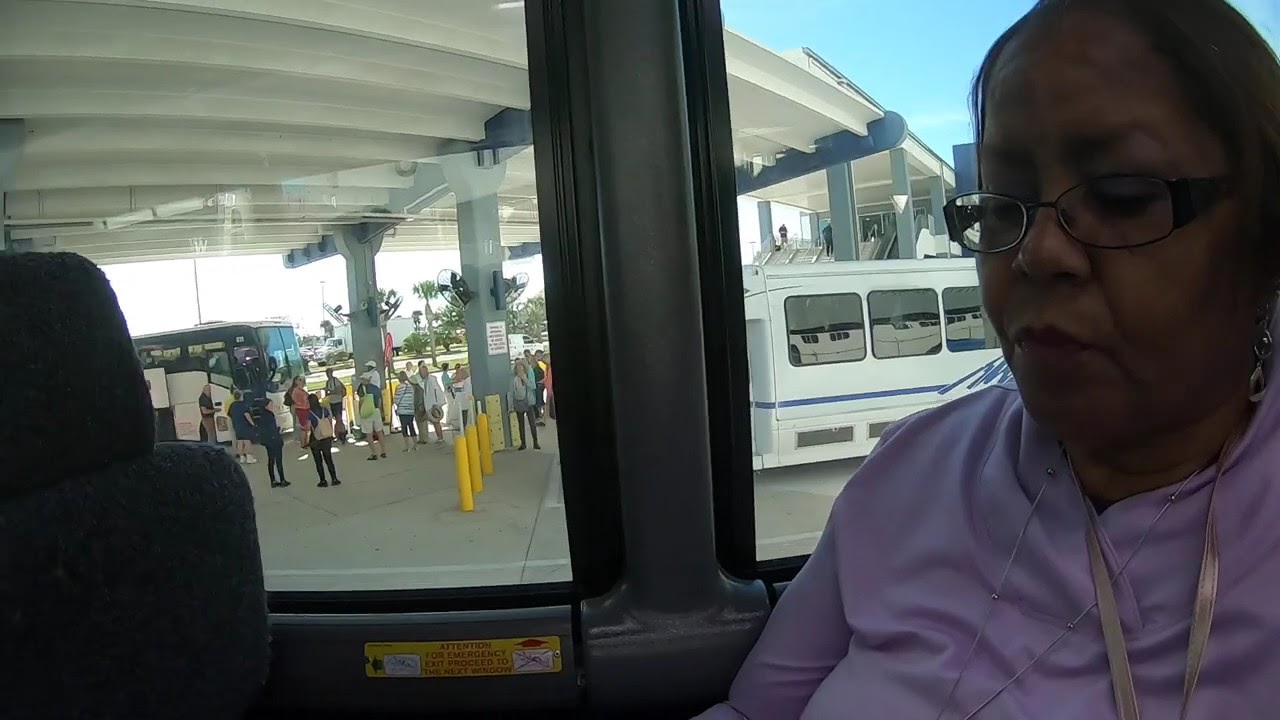In this photograph, taken from inside a bus or van, we see a vibrant scene that appears to be part of a transportation hub, possibly an airport terminal or bus depot. In the foreground on the right side, an older woman with dark skin and black glasses sits wearing a light purple jacket and a golden fabric strap around her neck. The bus is parked under an overpass, with a clear, sunny blue sky visible in the upper right corner. Through the large windows of the bus, we can see another van directly behind and a bus to the left. On the left side of the frame, groups of people mill about, possibly waiting for their own buses or other forms of transportation. The scene is bustling yet no clear signage reveals the exact location, leaving the precise nature of the hub open to interpretation.